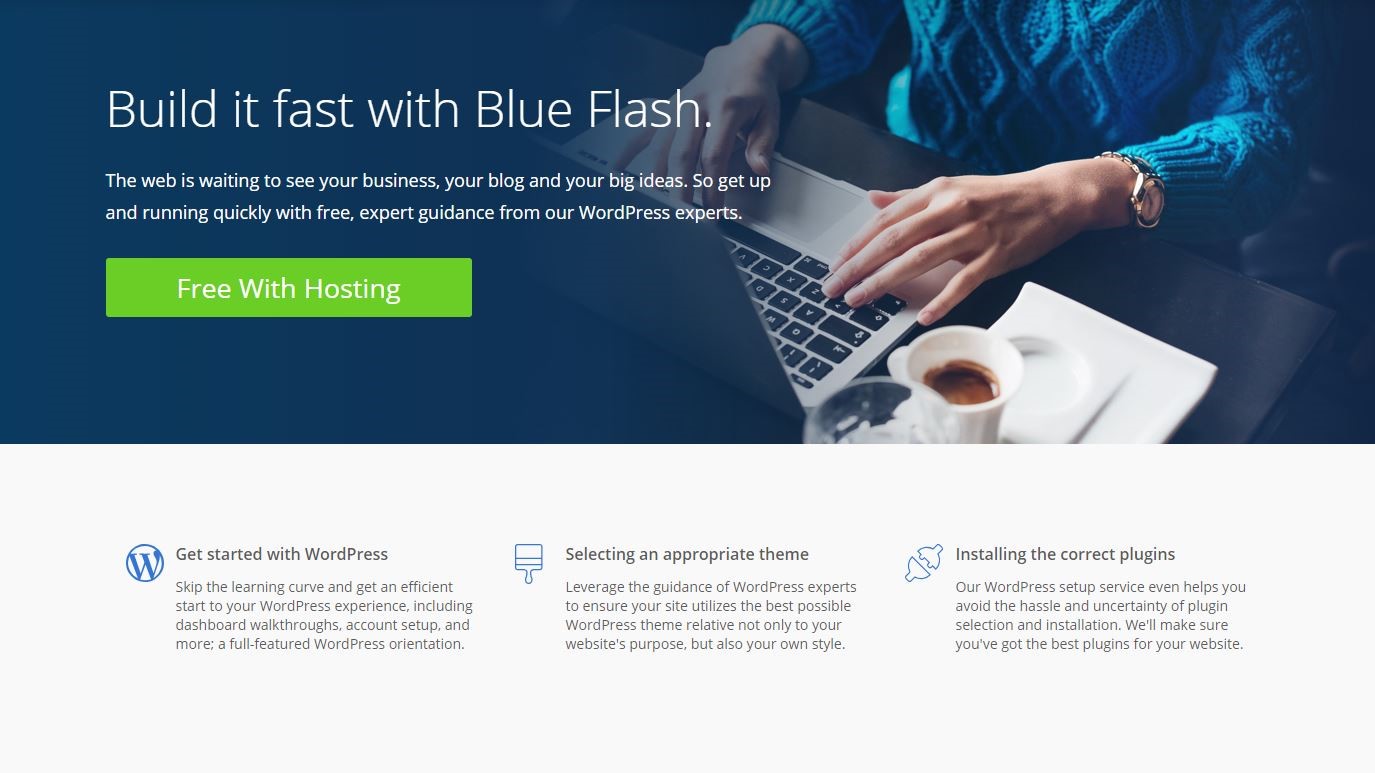The screenshot displays a hosting website interface. At the top, spanning from left to right, is a predominantly blue banner. Towards the right side of the banner, starting just before the center, there is a gradient transition to an aerial image of a woman working at a desk. The image, taken from a slightly tilted overhead angle, shows the woman’s hands typing on a laptop, revealing the laptop’s keyboard and the top of the screen. The woman's torso is visible, but her face is cut off at the top of the image.

In the banner, the text "Build it Fast with Blue Flash" is prominently displayed. Below this text, there is a green call-to-action button labeled "Free with Hosting." Just beneath the button, the text reads "Get Started with WordPress."

Underneath the banner, the page is divided into three side-by-side blurbs. The first blurb, titled "Get Started with WordPress," focuses on guiding users through the initial setup. The second blurb, "Selecting an Appropriate Theme," provides advice on choosing the right theme for their website. The third blurb, "Installing the Correct Plugins," offers tips on selecting and installing essential plugins.